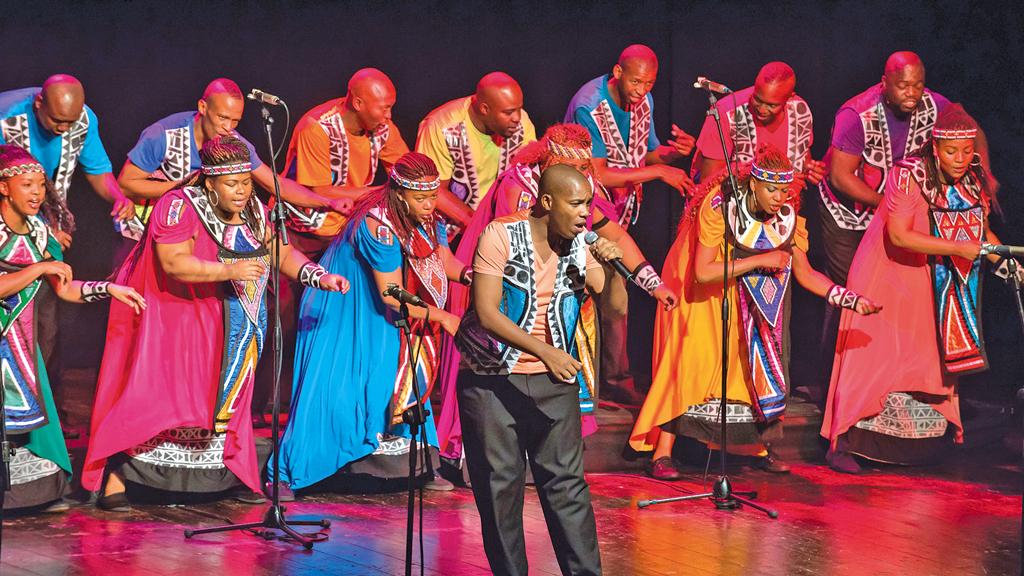The image depicts a vibrant stage scene featuring a male performer in the foreground and several background performers. The central figure is a man dressed in a tan t-shirt, dark pants, and a colorful vest adorned with black geometric patterns. He is leaning forward, singing into a microphone held in his left hand, while his right arm extends outward. Surrounding him are multiple microphones on stands, adding to the dynamic setup.

Behind him, there are two rows of performers, with the front row comprising women and the back row comprising men. The women are dressed in colorful robes with intricate headgear, showcasing hues of red, yellow, blue, and pink. The men are similarly attired in vibrant t-shirts, vests, and pants. Both rows of performers are leaning forward and appear to be mouthing or singing, harmonizing with the lead singer.

The stage is illuminated by an array of stage lights casting purple, red, and blue hues, which reflect vividly off the shiny floor, enhancing the overall colorful and lively ambiance. The background of the scene is dark, ensuring that the brilliantly dressed performers and their coordinated movements take center stage.